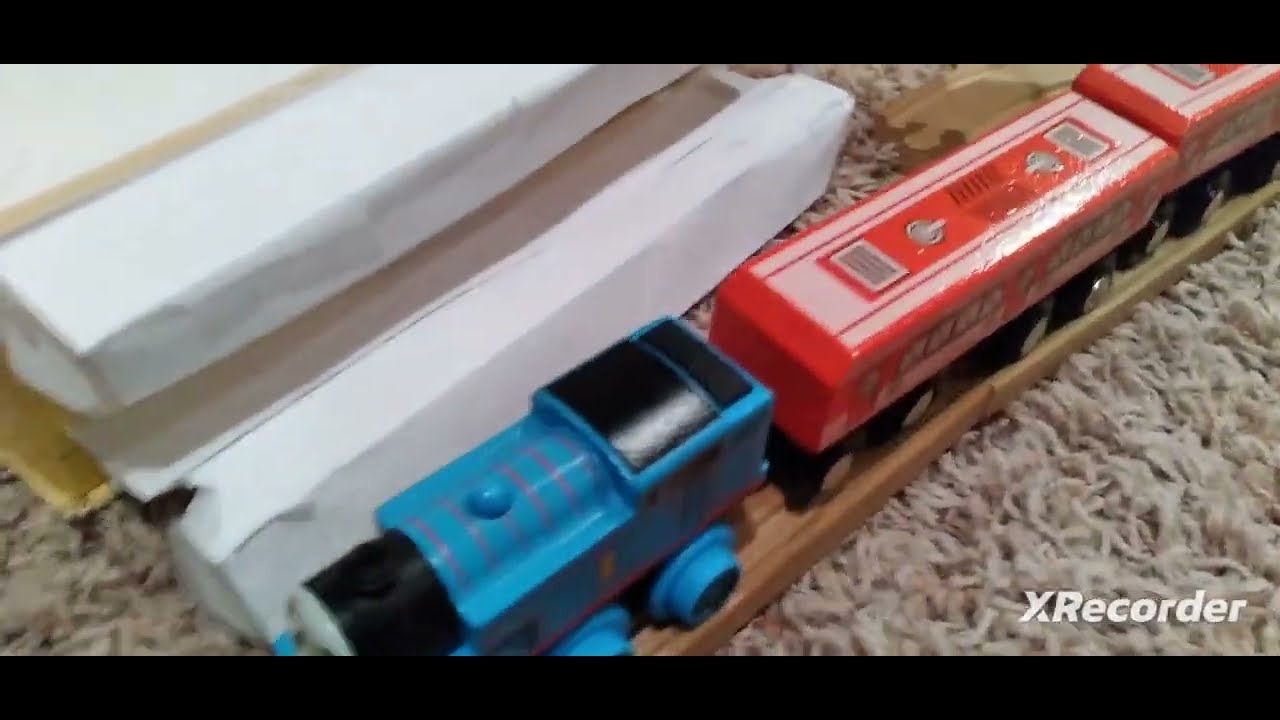The image depicts a detailed view of a toy wooden train set modeled after Thomas the Tank Engine from the children's show. The iconic blue and black engine features a grey face at the front and the number 1 on its side. Attached to Thomas are two red and white train cars, complete with detailed windows, doors, and panelling. The train, with its colorful carriages, is positioned on a wooden track with grooves, which lies on a beige, shaggy rug. In the upper left corner, the packaging materials can be seen, suggesting the train has been recently unpacked. The text "X Recorder" appears in the bottom right corner of the image. The photo captures an overhead perspective, showcasing the vibrant colors—blue, black, red, white, and touches of yellow and gray—of the toy train and its setting.